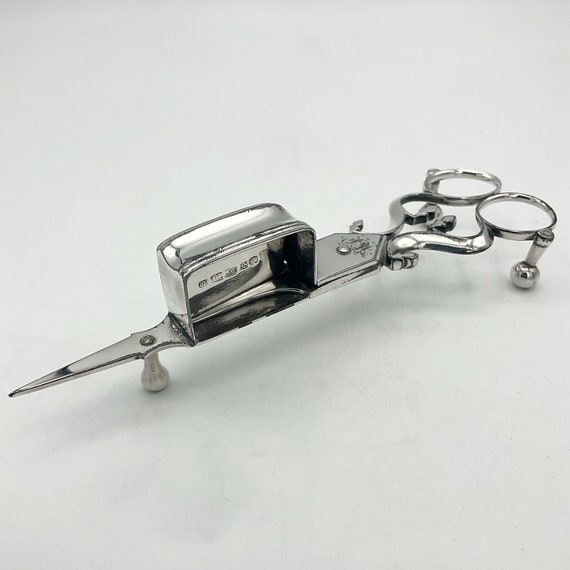This square image, approximately four inches by four inches, features a pair of unique scissors prominently placed against a light gray, almost white background. The scissors are positioned diagonally from the upper right-hand corner, where the handles rest, to the lower left, where the blades come to a point. The handles of the scissors, depicted in a metallic gray-black color, are on the upper right side, with the off-white background creating a stark contrast.

The silver, highly polished blades of the scissors reflect light, adding a notable shine to the image. Underneath the circles for the handles, small silver stands are attached, one supporting the scissors midway and another near the pointed end, lifting them slightly off the surface. At the top, where the blades meet, there is a raised metal piece resembling a toaster, the exact purpose of which is unclear. This detailed and meticulously arranged composition highlights the distinct features of the scissors, framed by the minimalist background.